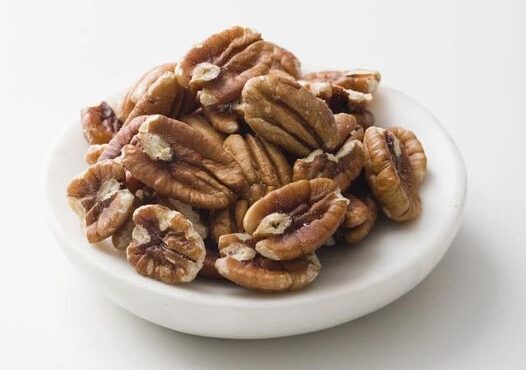This image features a shallow, white, slightly off-white plate holding approximately 20 pecan halves, situated against a white background. The plate's design includes a slight divot in the middle, resembling a bowl with very shallow sides, giving it a unique hybrid shape. The light brown pecans, distinctly without their shells, are strewn haphazardly across the plate, with some pieces displaying tan accents and vertical ridge lines, characteristic of their U-shape. There is a soft, subtle drop shadow under the plate, primarily on the lower right side, indicating gentle lighting. This detailed tableau emphasizes the delicate contrast between the pecans and the nearly blending hues of the plate and background.